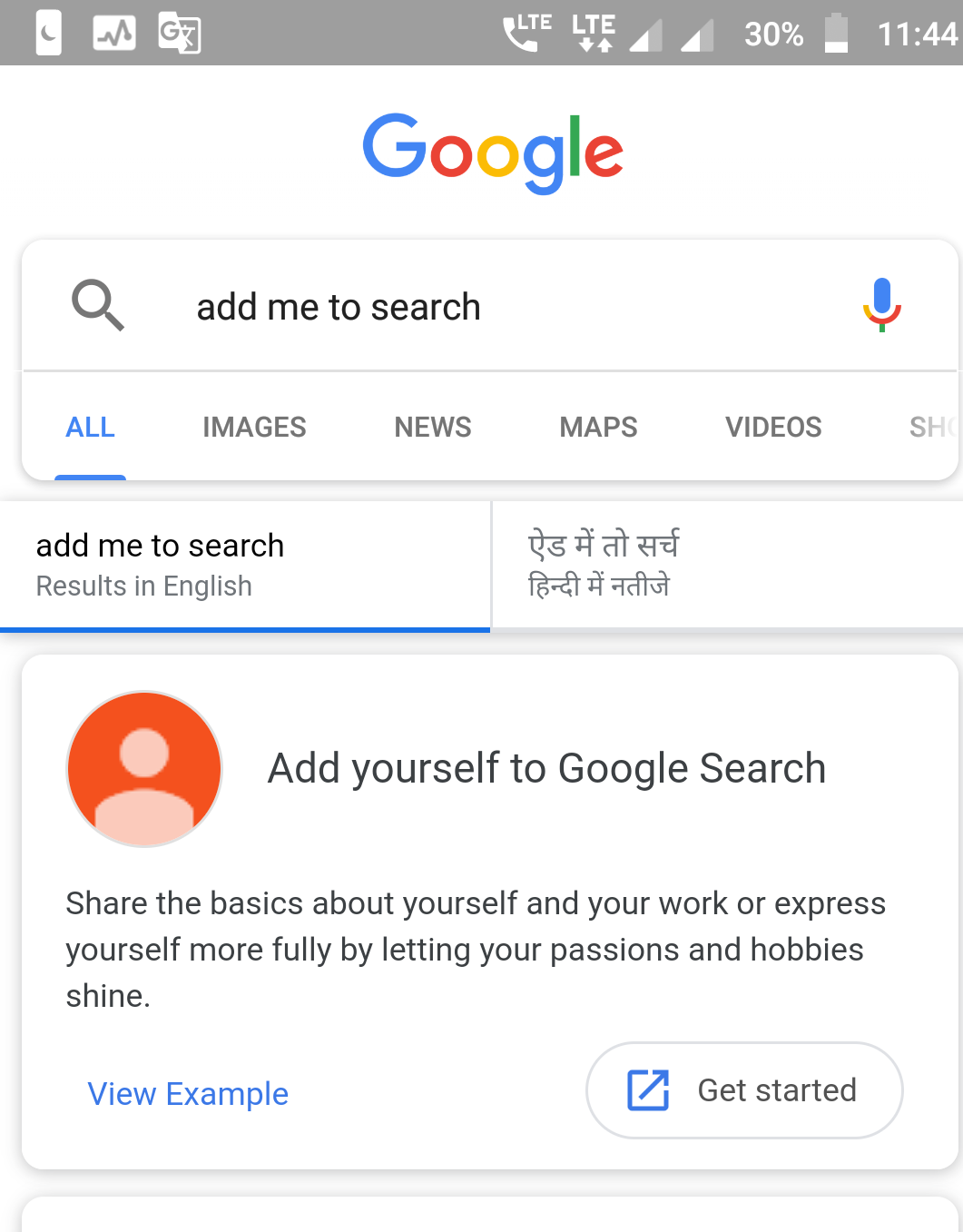The image depicts a digital interface resembling that of a computer tablet or smartphone screen, focusing primarily on displaying information.

At the very top, a dark gray banner spans across the screen, featuring a series of icons. On the left side of this banner, there are three small white icons, each enclosed in white rectangles. The center icon resembles a line graph. Another icon in the sequence is the letter 'G,' styled similarly to the Google logo. The upper right corner of the banner indicates the time as 11:44 and shows the battery level at 30%.

Below the dark gray banner, the background changes to white, prominently displaying the colorful Google logo. The logo consists of a blue capital 'G,' followed by lowercase letters: 'o' in red, 'o' in yellow, 'g' in blue, 'l' in green, and 'e' in red. Beneath the logo lies a search bar. Starting on the left inside the search bar is a magnifying glass icon, while on the right is a blue microphone icon. The placeholder text in the search bar reads "Add me to search."

Below the search bar is a navigation bar. The word "All" is highlighted in blue, suggesting it is the selected category. Other categories listed in dark gray or black capital letters include "IMAGES," "NEWS," "MAPS," and "VIDEOS."

Further down, two sections are displayed side by side. One section shows the text "Add me to search. Results in English." Next to it, a separate section contains text in a foreign language that is not legible or recognizable to the viewer.

At the bottom of the interface is a large rectangular banner prompting the user to "Add yourself to Google Search." Inside this banner is a prominent orange circle with an illustration of a person, depicted in a peach color, showing the head and torso.